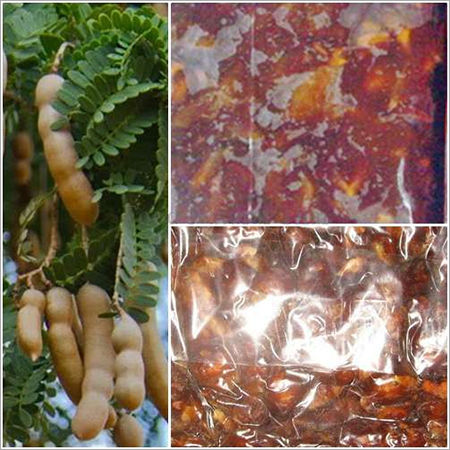The image depicts a distinctive plant on the left and packaged food products on the right. On the left side, there are clusters of green, oval-shaped leaves, from which elongated, beige, sausage-like pods emerge. These pods appear to have a hard outer shell, possibly containing seeds or nuts within. On the right side, several plastic bags or packets are filled with an unidentified red substance, seemingly marinated in a sauce or seasoning. The logical assumption is that the plant shown on the left is the source of the contents marinating within the plastic bags on the right.